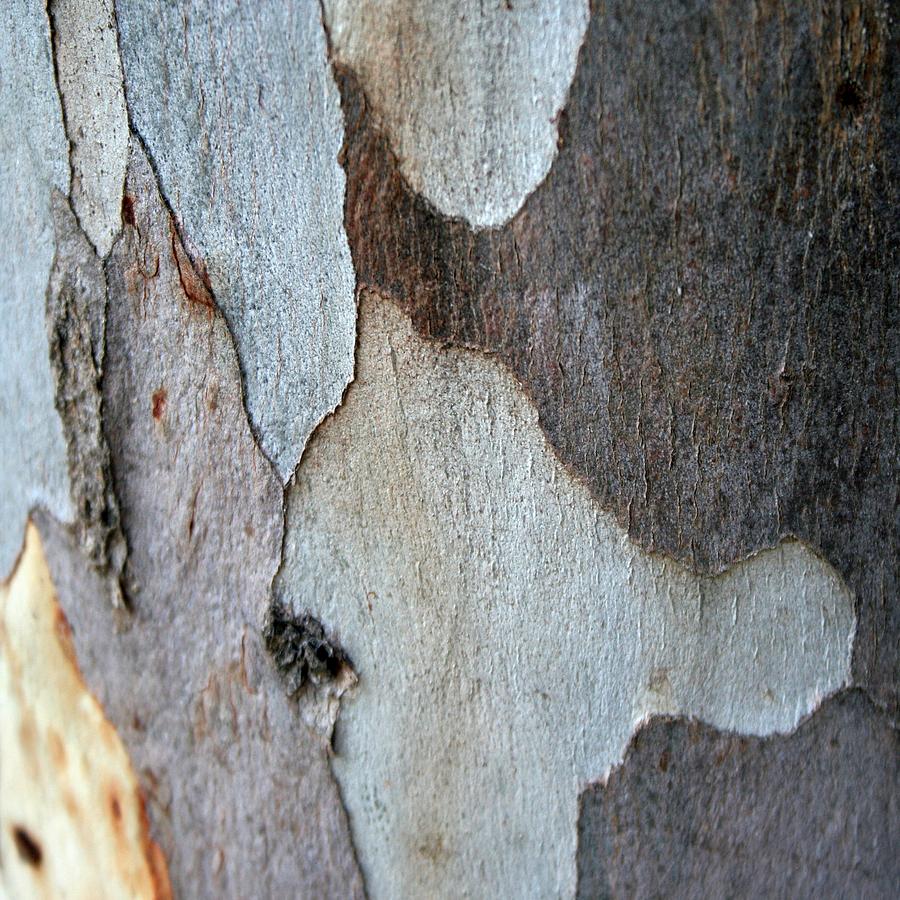This image is a close-up, highly detailed photograph of a tree trunk, showcasing the intricate and varied textures of its bark. The bark is discolored in different ways, giving the impression of an abstract pattern. In certain areas, the bark is missing, displaying underlying layers of the wood, which add to the complexity of the visual texture. 

On the left side of the image, there's a distinct yellowish area that resembles a flame, a stark contrast to the adjacent gray sections that look like icicles. These gray sections have blackish discolorations on their sides, contributing to the overall irregular and colorful pattern. 

The upper part of the image has patches of gray bark, while towards the right side, the wood transitions from dark brown to nearly black, marked by distinct knots and varied wood grain. The lower parts show lighter patches with a slate gray tinge of blue and light brown highlights.

This photograph, while abstract in its appearance, remains deeply rooted in the natural textures and variations of tree bark. Its artistic rendering captures the myriad colors and forms found in nature, making it a fascinating subject for close examination.